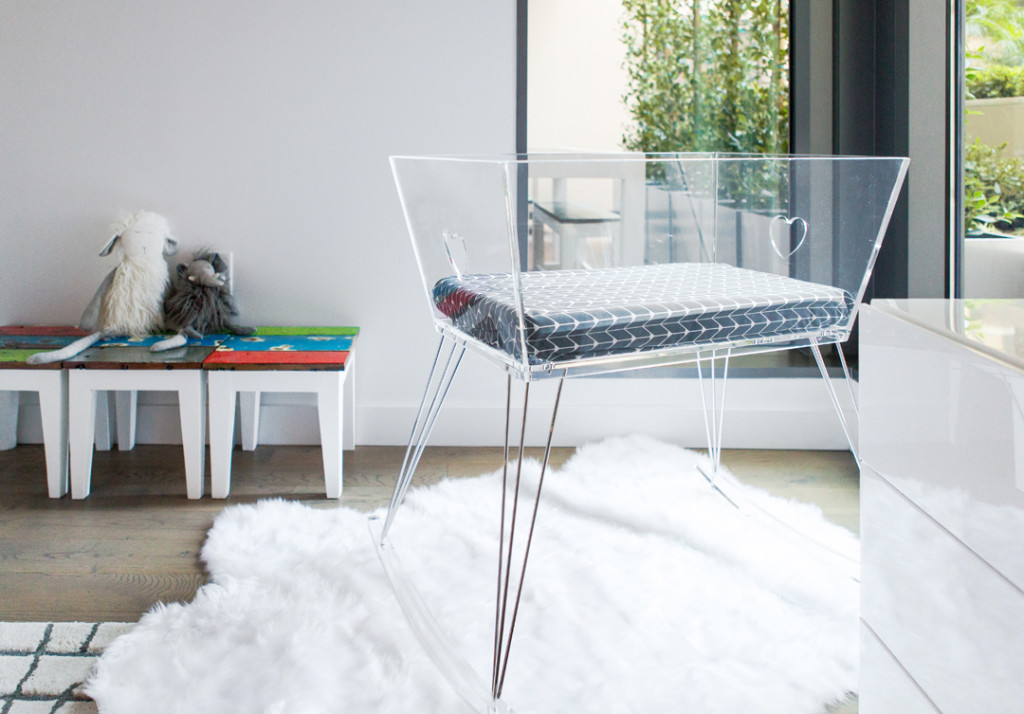The photo depicts a warmly lit, inviting children's room captured from eye level. Against the white wall, there are three cheerful, small benches with white legs and brightly colored tops, neatly arranged side by side. Adorning these benches are a few stuffed animals, adding a touch of playfulness to the space. To the right of the benches, a large window allows natural light to flood into the room. Just below the window stands a modern, translucent chair with sleek wire legs, positioned on a cozy sheepskin rug that adds texture and comfort to the wooden floor beneath. In the foreground on the right, partially visible, is a white cabinet of drawers, suggesting ample storage for a child's belongings. The overall ambiance of the room is one of warmth and playful charm, designed with both functionality and aesthetics in mind.